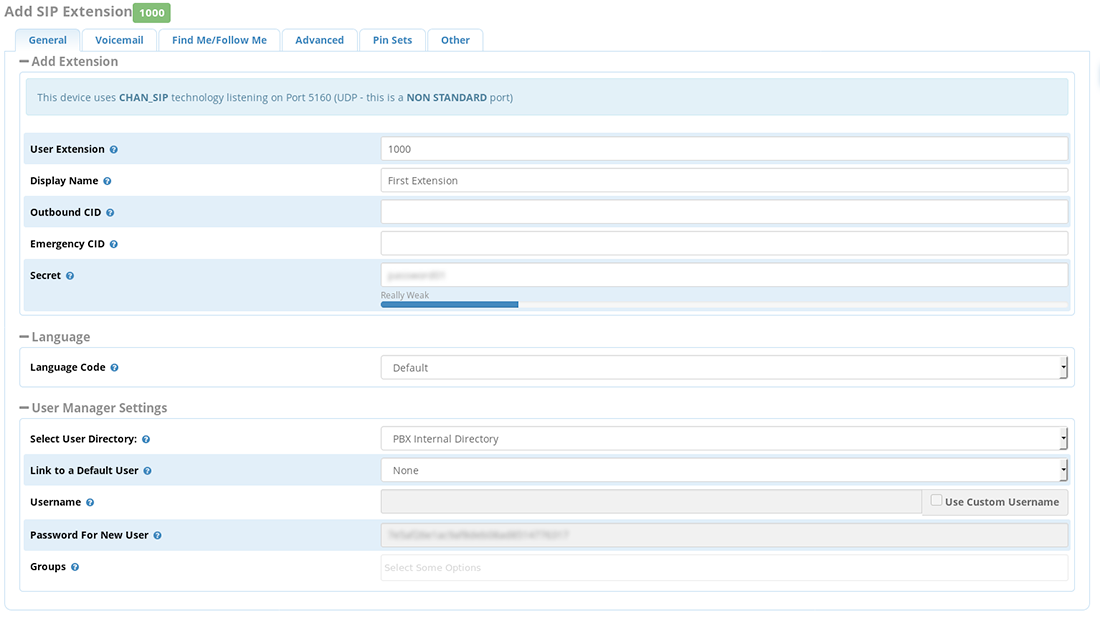The screenshot displays a web page interface of a software program for managing SIP extensions. At the very top, in black lettering, it reads "Add SIP Extension" with a small green box adjacent to the text marked "1000." Below this, there is a section with tabs, highlighted in blue text, labeled as: General, Voicemail, Find Me/Follow Me, Advanced, Pin Sets, and Other. Currently, the "General" tab is selected, revealing a series of input fields and drop-down menus.

Directly underneath the section of tabs, in black lettering, it states "Add Extension." The fields available in the "General" tab include: User Extension, Display Name, Outbound CID, Emergency CID, and Secret, each accompanied by a question mark icon indicating that these are options for the user to choose from via drop-down menus.

Further down, there is a "Language" section consisting of "Language Code" options. Following this, the "User Manager Settings" section allows for the selection of User Directory, Link to a Default User, Username, Password for New User, and Groups, with corresponding drop-down boxes to facilitate these selections.